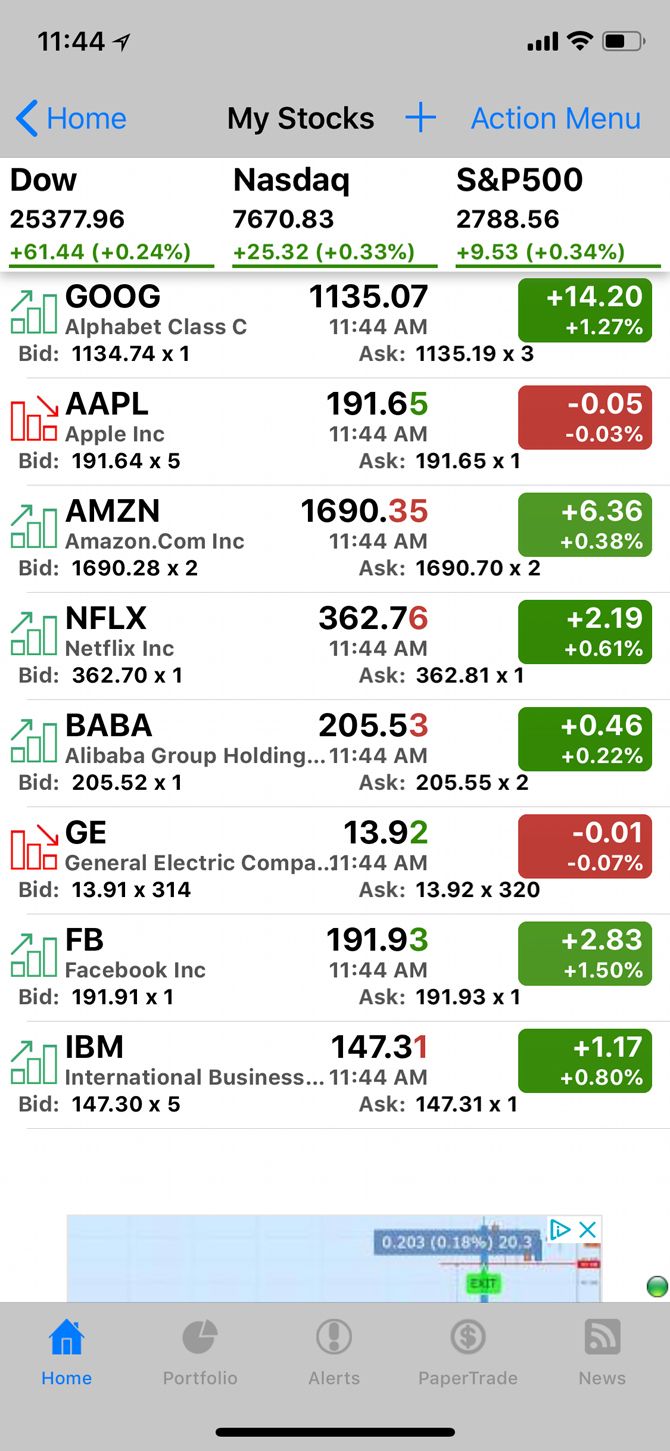The image depicts a detailed stock chart interface. Located at the top of the chart, the current time is displayed as 11:44. The status bar indicates full signal strength and Wi-Fi connectivity, while the battery is shown as half full. Directly below this, there are navigation indicators: a blue arrow with the word "Home" in blue digits, "My Stocks" in black digits, a blue plus sign, and "Action Menu" in blue digits.

Further down, three columns list major indices labeled in black letters: Dow, NASDAQ, and S&P 500. The Dow is recorded at 25,377.96, up by 61.44 points. The NASDAQ shows a value of 7,670.83, an increase of 25.32 points. The S&P 500 stands at 2,788.56, up by 9.53 points.

Beneath these indices, there is an extensive list of individual stocks accompanied by their respective ticker symbols and current prices:
- GOOG (Google): $1,135.07
- AAPL (Apple): $191.65
- AMZN (Amazon): $1,690.35
- NFLX (Netflix): $362.76
- BABA (Alibaba): $205.53
- GE (General Electric): $13.92
- FB (Facebook): $191.93
- IBM (International Business Machines): $147.31

The chart provides a comprehensive snapshot of current stock market conditions, complete with key metrics and individual stock performances.